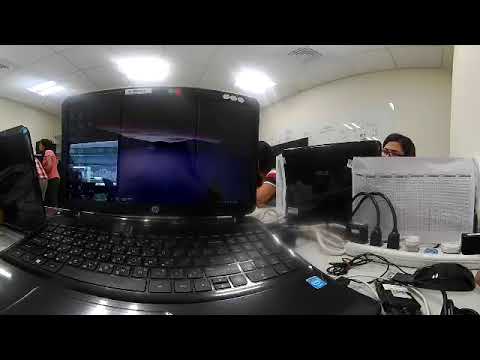The image captures a bustling office environment with a detailed view of a workspace. Dominating the center is a black HP laptop, its screen displaying what appears to be a videoconference. Surrounding the laptop are various office essentials, including a black mouse and a tangle of wires extending from an extension socket plugged into the wall. The workspace is cluttered but functional, hinting at a busy day.

In the background, multiple people can be seen engaged in their tasks. One prominent figure with brown hair and glasses is partially obscured by the laptop and a piece of paper resembling a white schedule. Another individual is wearing a pink shirt and jeans, while a third person sports a red and white plaid shirt. The presence of these colleagues adds a sense of community and collaboration to the scene.

The office itself features white walls and a white-paneled ceiling illuminated by fluorescent lights, contributing to a bright and efficient atmosphere. The overall setting suggests a typical modern office, where technology and human interaction blend seamlessly.